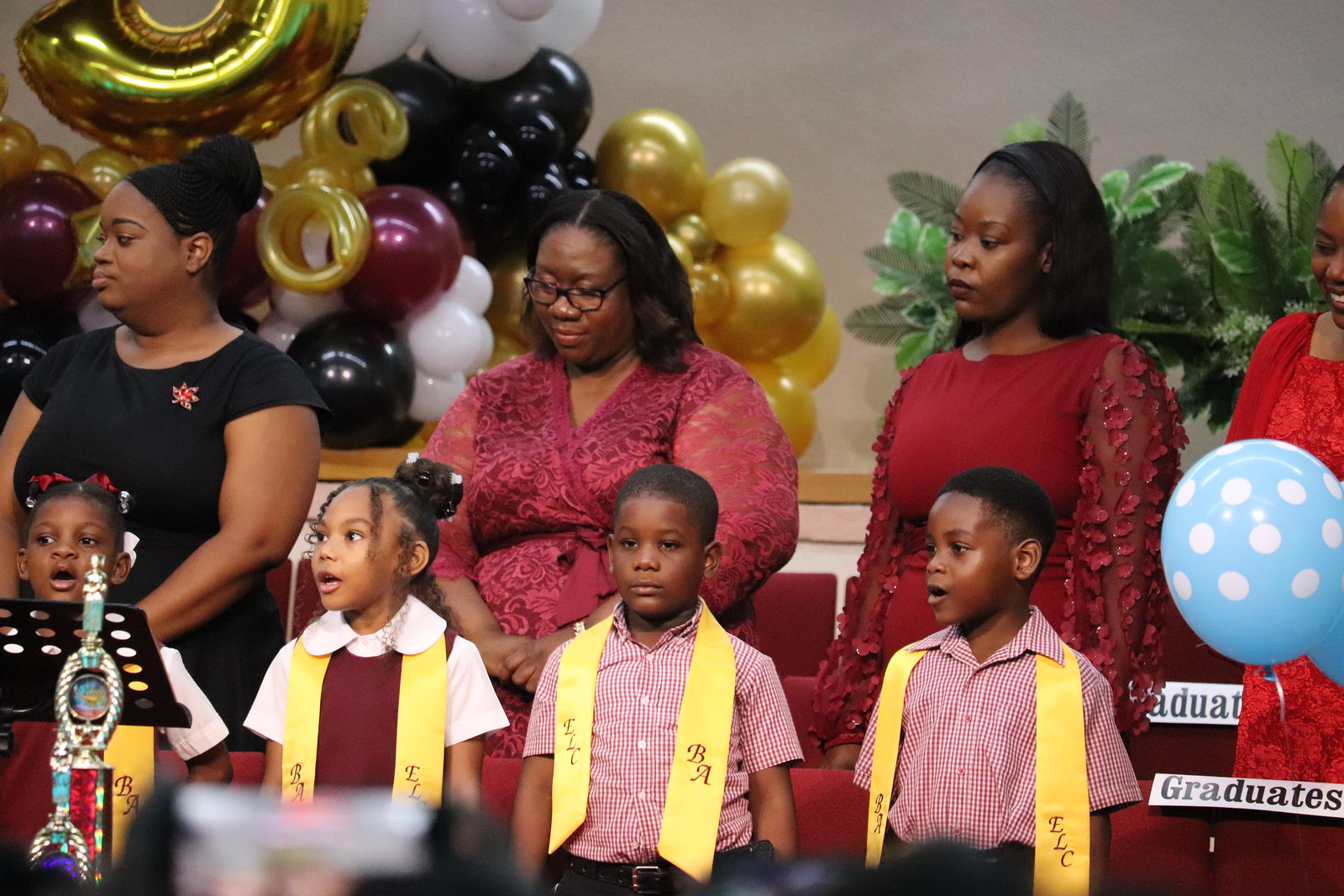The image depicts a lively indoor graduation ceremony, likely for young children from preschool, kindergarten, or first grade. The foreground features four young children—two boys and two girls—each adorned with a sash reading "ELCBA." The boys are dressed in blue and white checkered shirts, while the girls are wearing white shirts with red pinafores. Three of the children appear to be singing joyfully, while one boy stands nonchalant. Standing proudly behind them are four elegantly dressed African American women, presumably their mothers. The woman on the far right is in a red dress with a matching headband, the next woman sports a burgundy dress and glasses with her black hair down, and the woman on the far left is in a black top with her hair styled in a bun. The room is festively decorated with an array of balloons in blue, black, white, red, gold, and burgundy hues. Seats behind the children prominently display the word "graduates," underscoring the celebratory mood of the occasion.